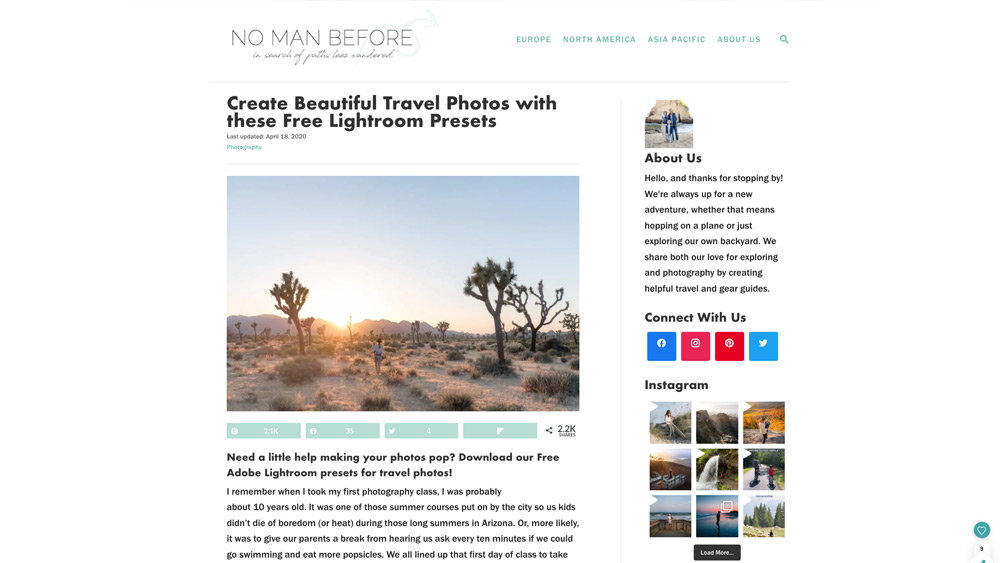The image features a clean white border at the top with gray text that reads "No Man Before." Below this, there is some cursive text that is too blurry to decipher. To the right, clear text reads "Europe, North America, Asia Pacific, About Us," and next to it, there's a magnifying glass icon, indicating a search function. Beneath this section, there is a gray line followed by the text, "Create beautiful travel photos with these free Lightroom presets."

The main image appears to showcase Joshua Tree National Park under a stunning blue sky. The sun is either rising or setting behind a range of mountains, casting a warm glow over the sparse, scrubby vegetation typical of the area. Several iconic Joshua trees are scattered throughout the scene, and a lone hiker is captured in the middle of the photograph, adding a sense of scale and adventure.

Below this captivating landscape, the text reads, "Need a little help making your photos pop? Download our free Adobe Lightroom preset for travel photos." On the right side of this section, there are options to connect with the brand via four different social media links.